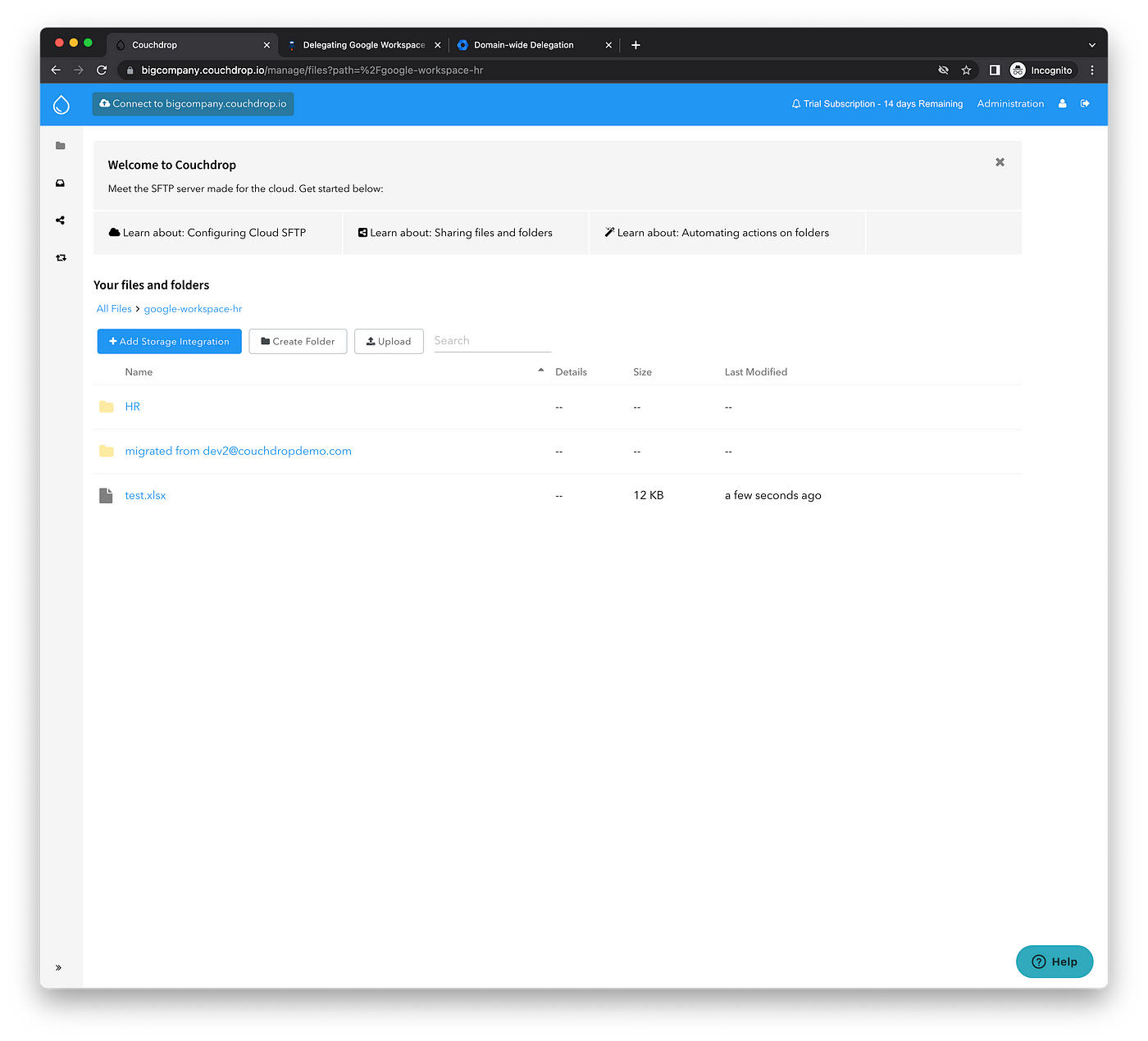The image is a screenshot with a somewhat blurry quality. In the top left corner, there are three colored circles—red, yellow, and green—likely representing the window control buttons of an operating system. There are three browser tabs open; the active tab is titled "CountDrop." The other two tabs are labeled "Delegating Google Workspace" and "Domain-Wide Delegation."

Below the tab bar, the web address visible is "Connect to BigCompany.CountDrop.io." The main content of the page starts with a bold heading that reads "Welcome to CountDrop." A subheading follows, stating: "Meet the SFTP server made for the cloud. Get started below."

The page continues with several informational links:
- "Learn about configuring cloud SFTP"
- "Learn about sharing files and folders"
- "Learn about automating action on folders"

Further down, there is a section titled "Your Files and Folders" with subcategories like "All Files" and "Google Workspace." Additionally, there are two prominent buttons labeled "Add Storage Integration" and "Create Folder."